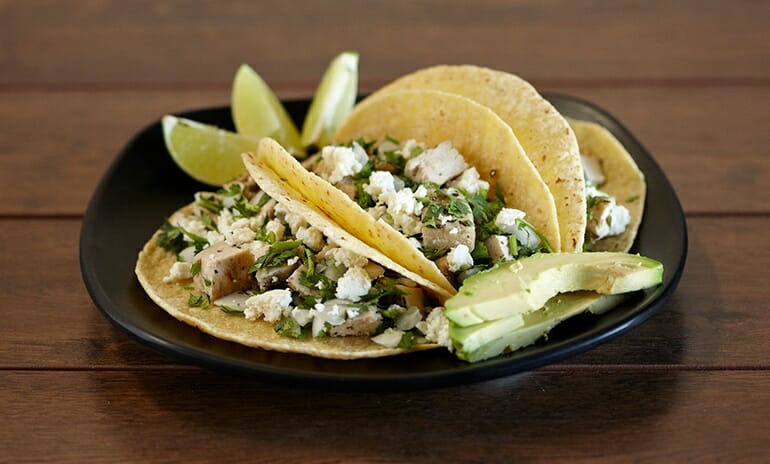This image features a professional-quality photograph of a black plate resting on a darker brown wooden table, composed of four distinct horizontal planks. The plate is the focal point and contains three tacos in crunchy shells, filled with diced chicken, fresh cilantro, and crumbly white cheese. Accompanying the tacos are a few slices of light green avocado and three green lime wedges, perfectly positioned for squeezing. The tacos and their accompaniments are front and center, dominating the frame with vibrant colors and appetizing presentation.